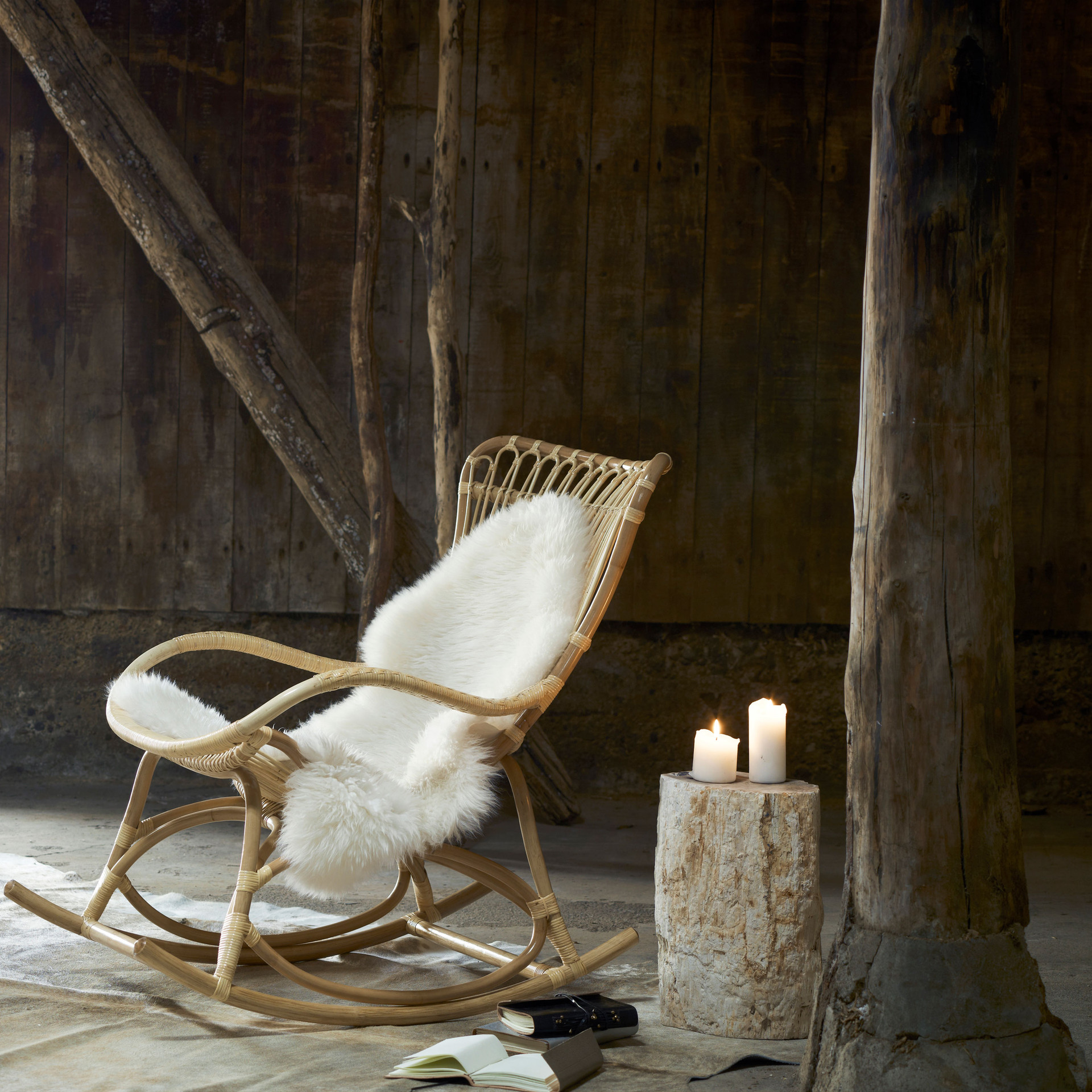In a rustic, barn-like room, characterized by wooden barn doors and support beams, this square-cropped image centers on a light wood, wicker rocking chair facing the left. The chair is adorned with a luxurious white fur throw, serving as a plush seat cover. Adjacent to the chair is a side table crafted from the trunk of a tree, painted an off-white shade. Atop the table, there are two lit candles, one short and round, the other tall and slender, casting a warm glow. The scene suggests a moment of interrupted reading, with three books scattered on the rough, tan rug that covers the wooden floor—one open and two closed. The lighting in the image highlights the white fur throw and the candle-lit tableau, while casting shadows in the corners of the room, adding to the rustic charm.